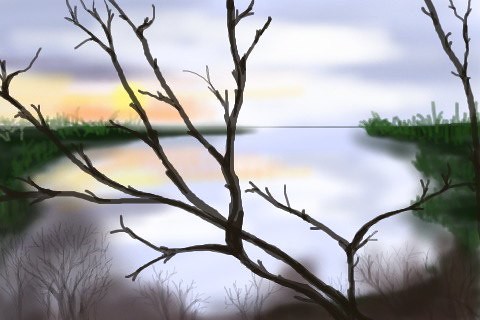The image is a computer-generated, animated depiction of a small, undulating pond surrounded by nature in what appears to be the fall or winter. The pond reflects a sky in various shades of gray, with hues of orange and yellow suggesting either a sunrise or sunset. Overhead, the sky is cloudy and slightly hazy, except where the sun breaks through. Surrounding the pond are green grass and tall, leafless trees with thin branches, indicating colder seasons. The water in the pond mirrors the color palette of the sky, adding depth to the scene. The horizon in the background remains misty, enhancing the tranquil, almost ethereal atmosphere of the artwork.